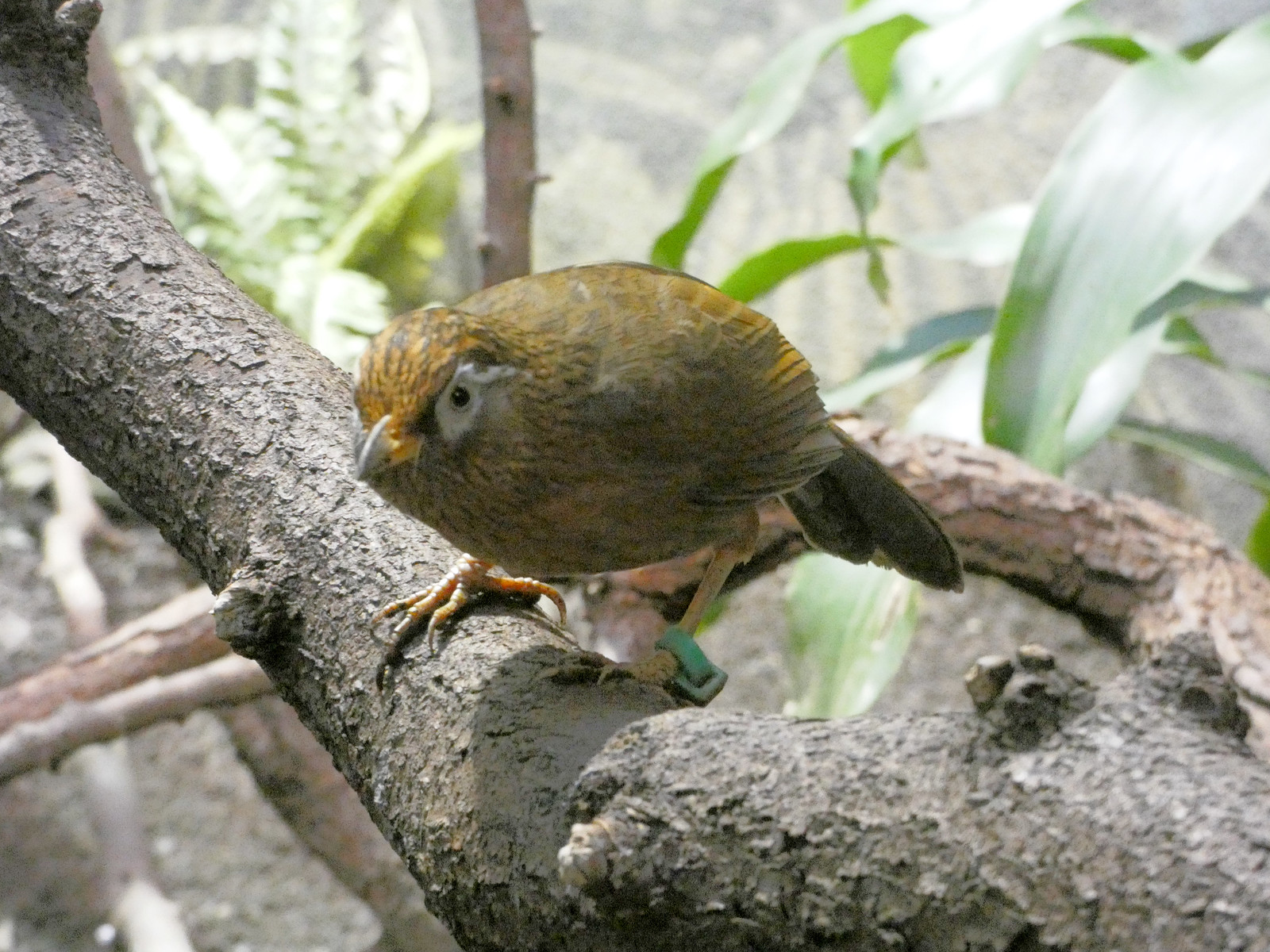The image captures a vibrant outdoor scene on a bright day. Dominating the foreground is a thick, rough-textured brown branch, with patches that appear whitish, possibly due to the sunlight highlighting the grainy bark. Perched on this branch is a bird that resembles a sparrow but is slightly larger. This bird has a predominantly brown body with hints of orange running through its feathers, particularly noticeable on its crest and wings. Its beak starts off gray near the head but transitions to an orange hue towards the body. The bird's black, beady eyes are accentuated by white rings around them. A green band is affixed to its left leg, suggesting it has been tagged for tracking purposes. The bird's claws grip the branch, and its orange feet are clearly visible. Surrounding the branch is lush greenery, with various green leaves and a fern noticeable in the top left corner. The background is illuminated by the sun, which casts a bright, white light throughout, adding to the image's natural, lively atmosphere. In the lower area, patches of dirt contrast with the vivid green of the plants, completing this detailed depiction of a serene outdoor setting.